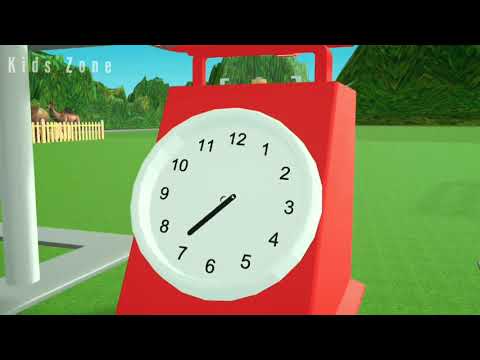The image appears to be a still shot from a digital animation or video game, portraying a cartoon-like scene. Dominating the left-hand side of the background is a clear blue sky, extending seamlessly across the top. To the right-hand side, a simplistic triangular green hill or mountain rises from the landscape, partially bordered by a line of green trees or shrubbery. Below, a wide expanse of flat, uniformly green grass stretches out, giving a simple, almost artificial look without any individual blades standing out.

In the upper left-hand corner of the image, the text "Kids' Zone" is displayed in bold white font, set against a dark border that runs horizontally across the top and bottom of the screen. A wooden fence section can be seen on the left-hand side, enclosing an area that visually contains what seems to be camels or horses. Just in front of this fenced area stands a white pole anchored to a white square base.

The foreground is dominated by a prominent red object reminiscent of a weight scale. This scale features a white circular face marked with black numbers from 1 to 12, bearing a single black pointer that indicates a position just past 7. The scale’s design is peculiar, with its top slanting forward slightly, and supported by two red poles extending from its upper section. The overall setup, combined with the simple and vibrant colors, suggests an intentionally stylized and playful environment.